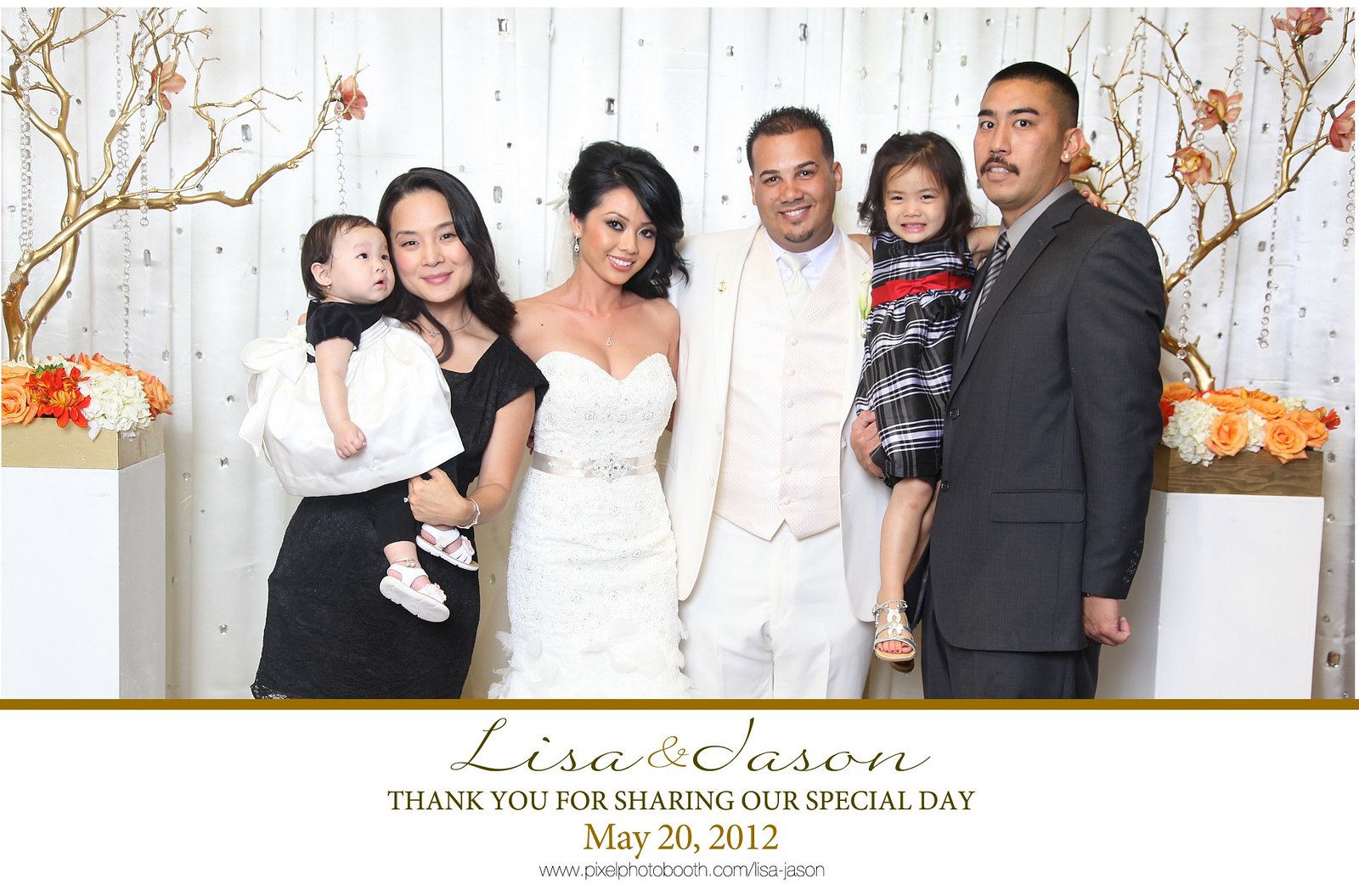The image is a professionally taken wedding photo card featuring a central family portrait against a background that mixes white curtains embellished with crystal-like decorations and a wooden setting. The people in the photograph are positioned in front of white pedestals adorned with orange and white flowers, accented by gold-painted tree branches. The groom, dressed in a white three-piece suit, stands beside the bride, who is in an elegant wedding gown. To their left is a woman in a black dress holding a baby dressed in black. To their right is a man in a dark suit holding a child, approximately four or five years old, who is wearing a black and white plaid dress with a red bow around the waist. Below the photo, on a white background with gold text, the card reads, "Lisa and Jason, thank you for sharing our special day, May 20, 2012." The URL "pixelbooth.com Lisa-Jason" is also displayed prominently, written in a darker color. The overall color scheme includes white, gold, black, red, orange, tan, gray, and various shades of brown, creating a harmonious and festive composition.